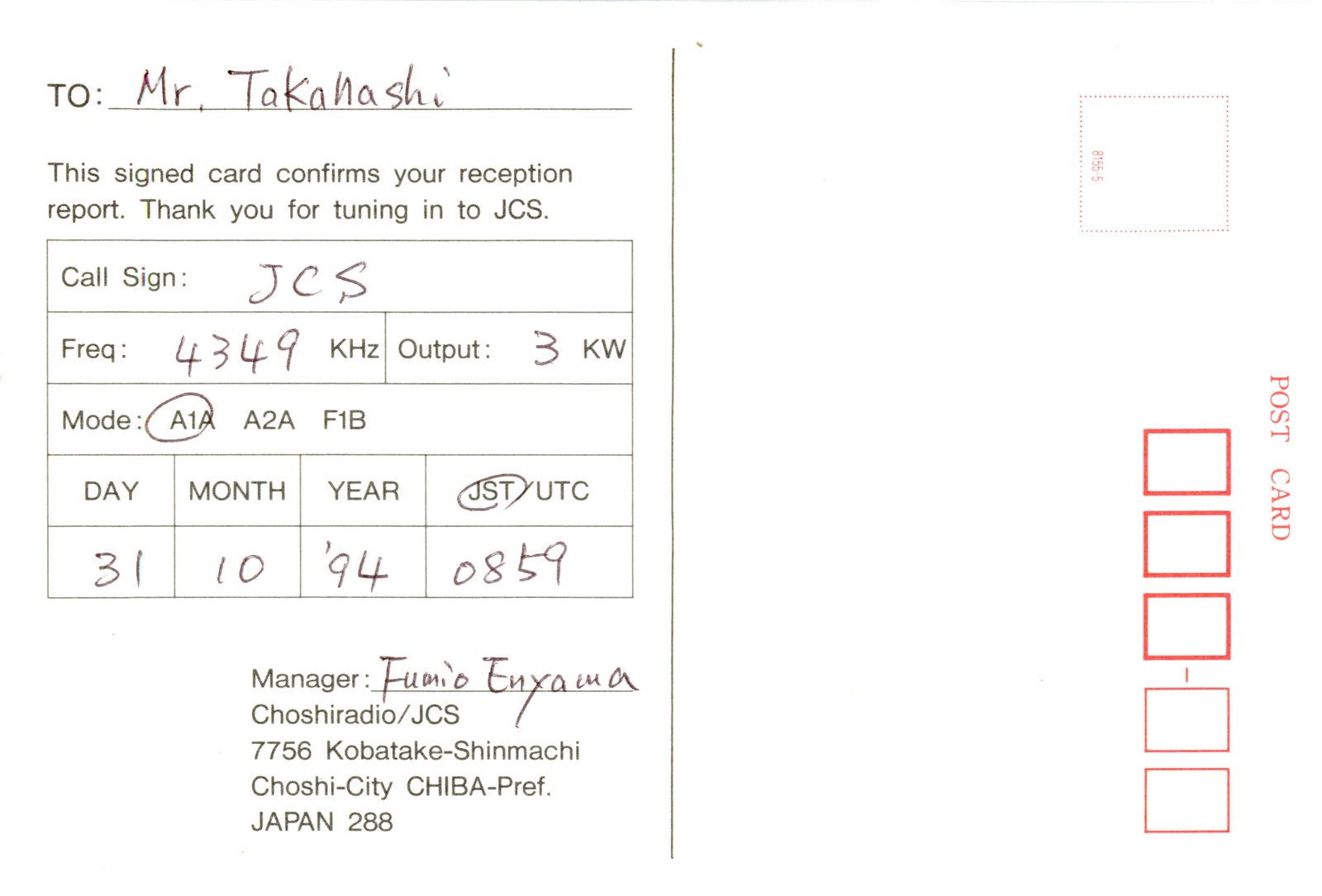This image showcases the back of a postcard with a printed reception report that has been filled in by hand. On the left side, the text addresses Mr. Takanashi and states: "This signed card confirms your reception report. Thank you for tuning in to JCS, call sign JCS, frequency 43.49 kHz, output 3 kW, mode AIA (circled instead of A2A or FIB), date 31/10/94, JST (circled) / UTC not circled, and time 0859." The report is signed by manager Fumio Enyamana with the address "Chiri Shiraito / JCS 7756, Kobatake Shinmachi, Kyushu City, Chiba Prefecture, Japan, 288." The background is primarily white with blue text, accented by red boxes. The postcard is visually divided in half vertically, with the detailed information on the left and five vertically aligned red squares plus the word "postcard" on the right. The top right features a blank space presumably for a stamp.